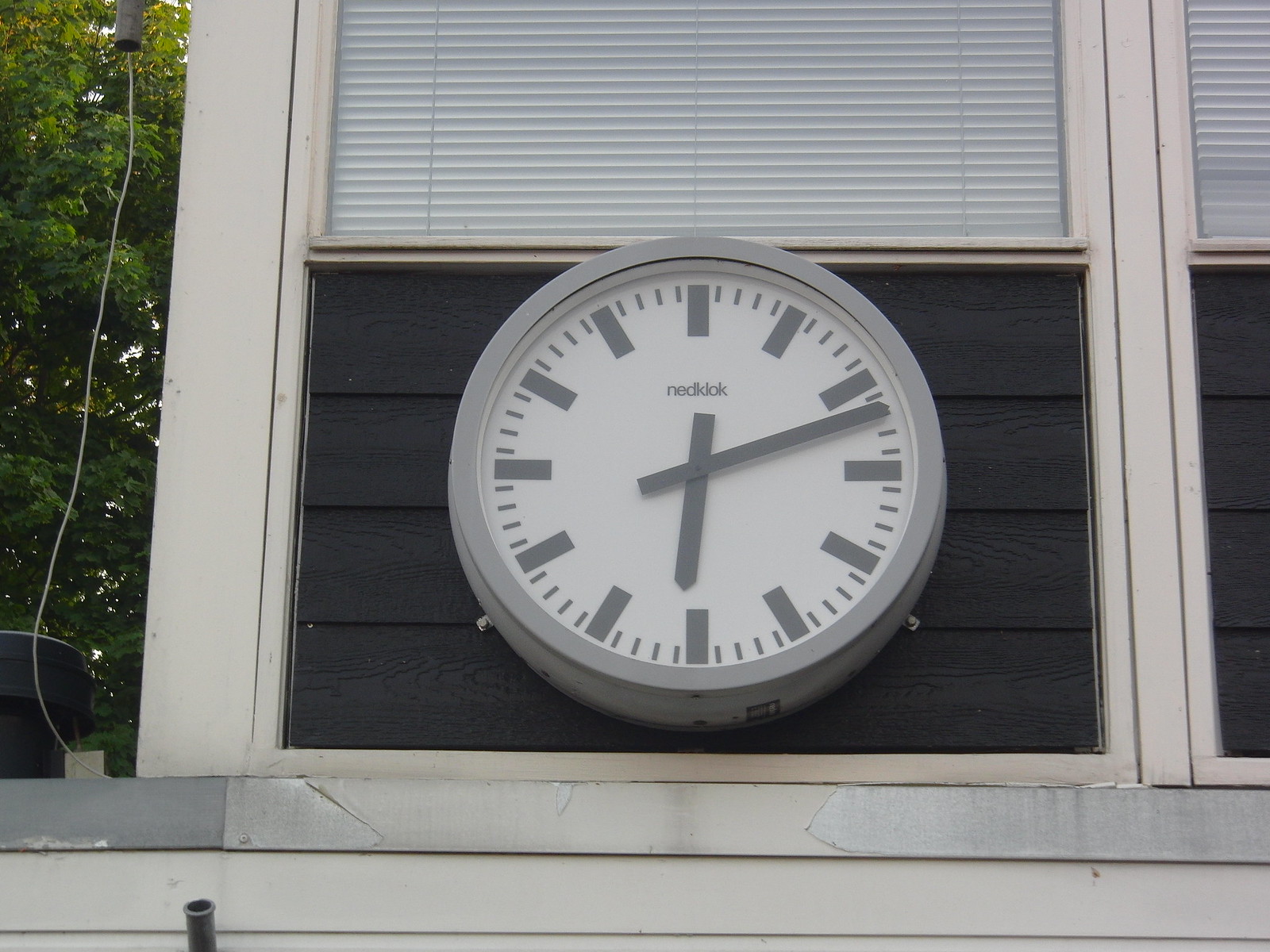The image depicts a large, round clock with a grey frame mounted on the side of a building just below a window. The clock, made of plastic, features grey notches in place of numbers and grey hands with dull pointers. It is bolted to wooden planks, which are painted black or very dark, and these planks are themselves attached to the building. Below these black planks, the building's siding is made of brown wood. The window above the clock has white blinds on the inside and white framing. In the upper left corner of the image, green leaves from nearby trees are visible, illuminated by sunlight. Additionally, a small pipe with a cable extends from above to the left side of the clock.